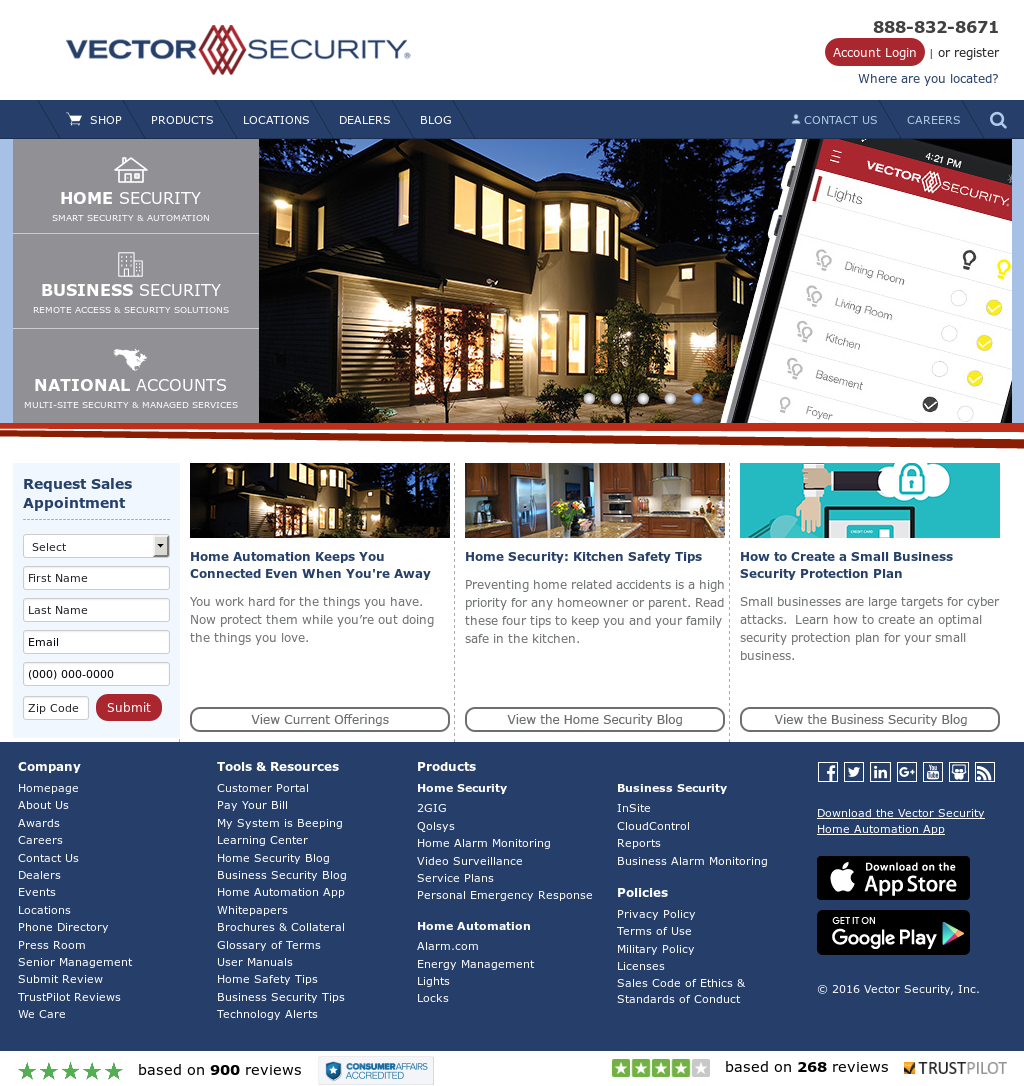In this image, the screenshot is set against a clean white background. In the upper left corner, the company website is prominently displayed in blue text alongside a red logo consisting of three red diamonds, representing Vector Security. In the upper right corner, a phone number, 888-832-8671, is clearly visible, accompanied by a striking red action button with white text that reads "Account Login or Register" and a prompt asking "Where Are You Located?"

Below this, a blue banner spans the width of the image, containing a navigational menu from left to right: "Shop" with a white shopping cart icon, "Products," "Locations," "Dealers," "Blog," "Contact Us," and "Careers." Additionally, there is a magnifying glass icon for search functionality on the far right.

The main section of the screenshot features a large, vibrant color photograph of a beautiful two-story home illuminated in a night scene, with all its windows brightly lit, giving a warm and inviting appearance.

At the bottom of the screen, five green stars indicate a stellar rating based on 900 reviews, whereas to the immediate right, there is a visual indicating a four out of five stars rating from Trustpilot.